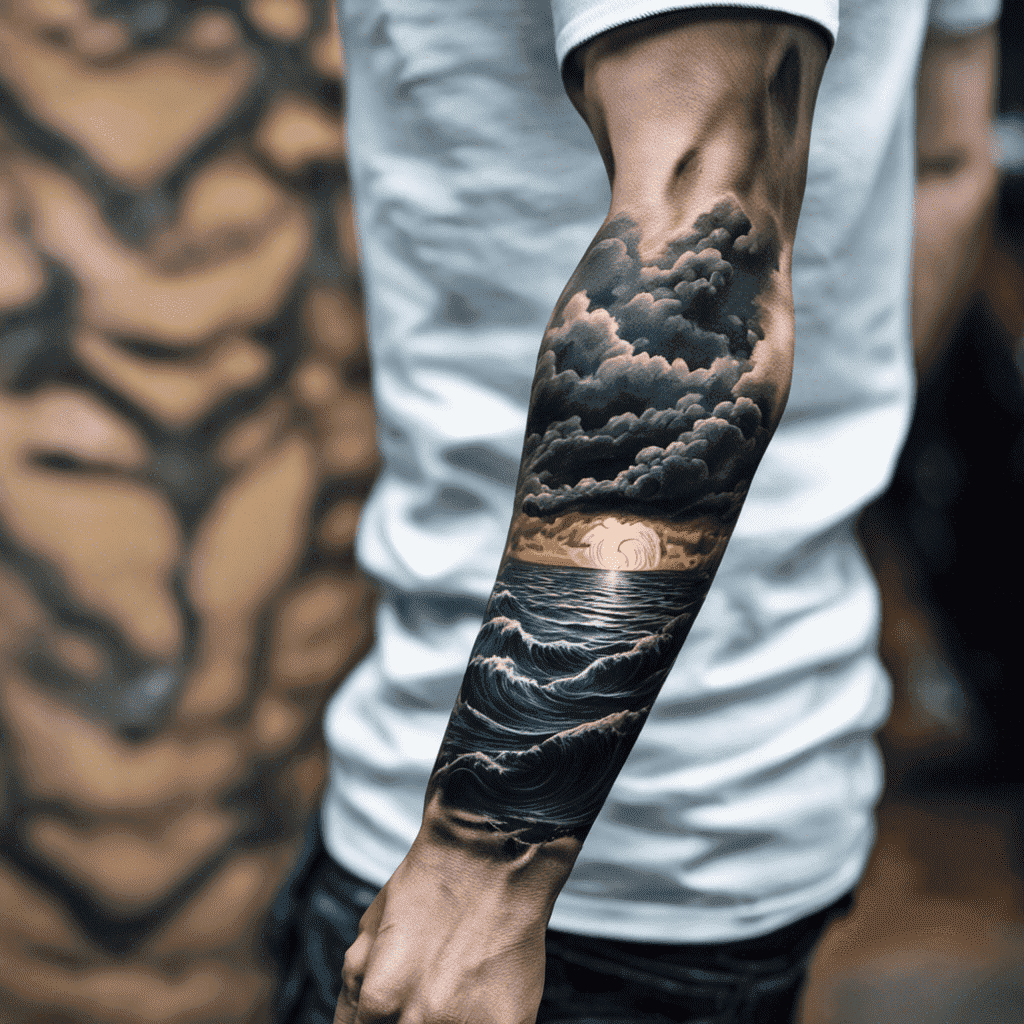The image features a lean, muscular man standing in front of a blurred, tan and black backdrop, which appears to have a veined pattern. He wears a slightly rumpled, white t-shirt that is too long, paired with dark jeans. The main focus of the highly saturated image is his tattooed right arm, which he is flexing slightly, revealing well-defined muscles and minimal hair. The intricate black and white tattoo spans from his wrist to just above his elbow and depicts a seascape masterpiece: dark clouds at the bottom transitioning to lighter shades at the top, large waves rippling across the ocean, and an open space of natural skin illustrating the sun amidst the clouds and waves. The contrasty image emphasizes the deep, dark colors and detailed artistry of the tattoo, making it the prominent feature against the indistinct background.